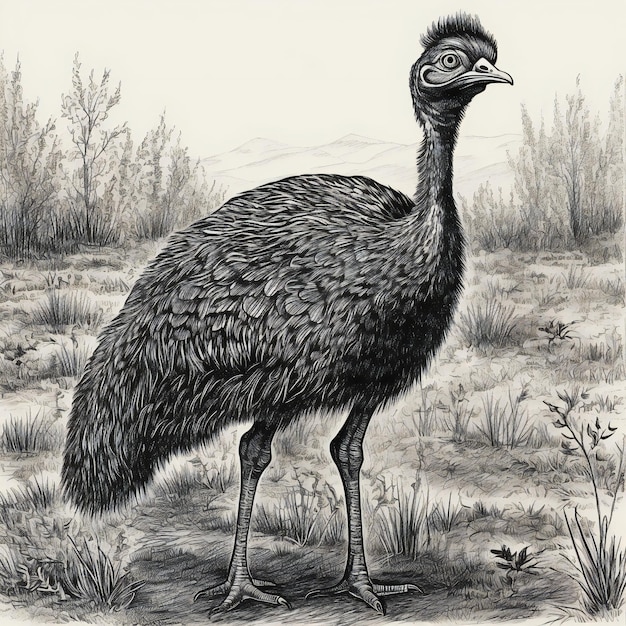This detailed black-and-white drawing on a white piece of paper features a prominent bird as its central figure. The bird, possibly a heron or crane, boasts a long, elegant neck adorned with a distinctive tuft of black feathers that stand upright atop its head. A noteworthy teardrop-shaped marking is situated just below its sharp beak, adding an intriguing element to its face. The bird's plumage consists of meticulously drawn layers of gray feathers that give it a textured and life-like appearance. Its slender, elongated legs are firmly planted in an expansive field brimming with grass and various weeds. The background of the illustration reveals several barren trees, contributing to a somewhat stark but serene landscape. A gently rolling hill completes the scene in the distance, adding depth to this beautifully detailed nature setting.